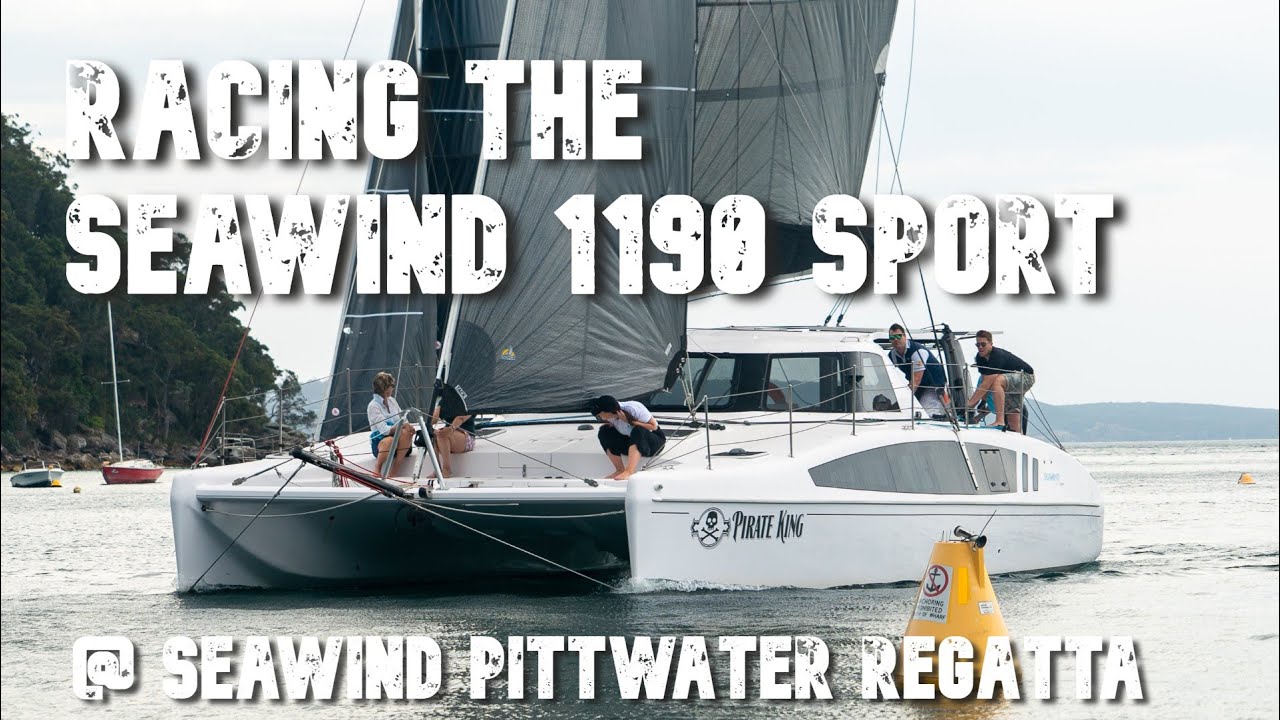This detailed image captures a dynamic scene featuring a boat named "Pirate King," identified by its prominent skull and crossbones logo on the side. The photograph, bright and taken during the daytime, shows a wide boat brimming with young people. Positioned towards the front are three individuals, while two men are situated near the steering area at the back. Text in large, worn block letters overlays the image, reading, "Racing the Sea Wind 1190 Sport" at the top and "at Sea Wind Pit Water Regatta" at the bottom. Towards the bottom right of the image lies an orange buoy with a barely discernible warning sign resembling an anchor crossed out. In the background on the left, two additional boats—one blue with a yellow section and one red—are visible, set against a backdrop of numerous trees and distant hills on the horizon. The overall scenery is well-lit and suggests vibrant, lively racing action on a beautiful waterway.